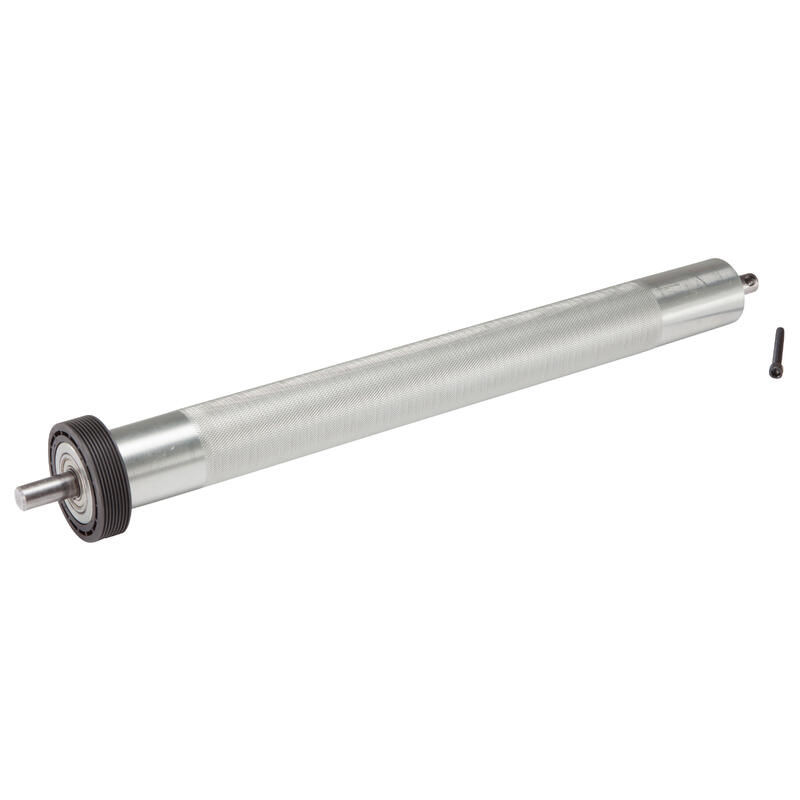The image features a single silver cylindrical piece of equipment, possibly resembling a bike pump, positioned flat and diagonally across the center against a completely white background. The object has a shiny silver surface at both ends, while the middle section exhibits a rougher texture. On the left end, a round black circle with thin black lines along its edges encases a central silver area, and a thin silver piece protrudes through its center. On the right end, another thin silver piece extends outward, accompanied by a small, vertically-standing dark gray screw-like component situated in front of the cylinder. The photograph, devoid of any text, highlights a color palette of white, silver, gray, and black, presented in a style typical of product listings.